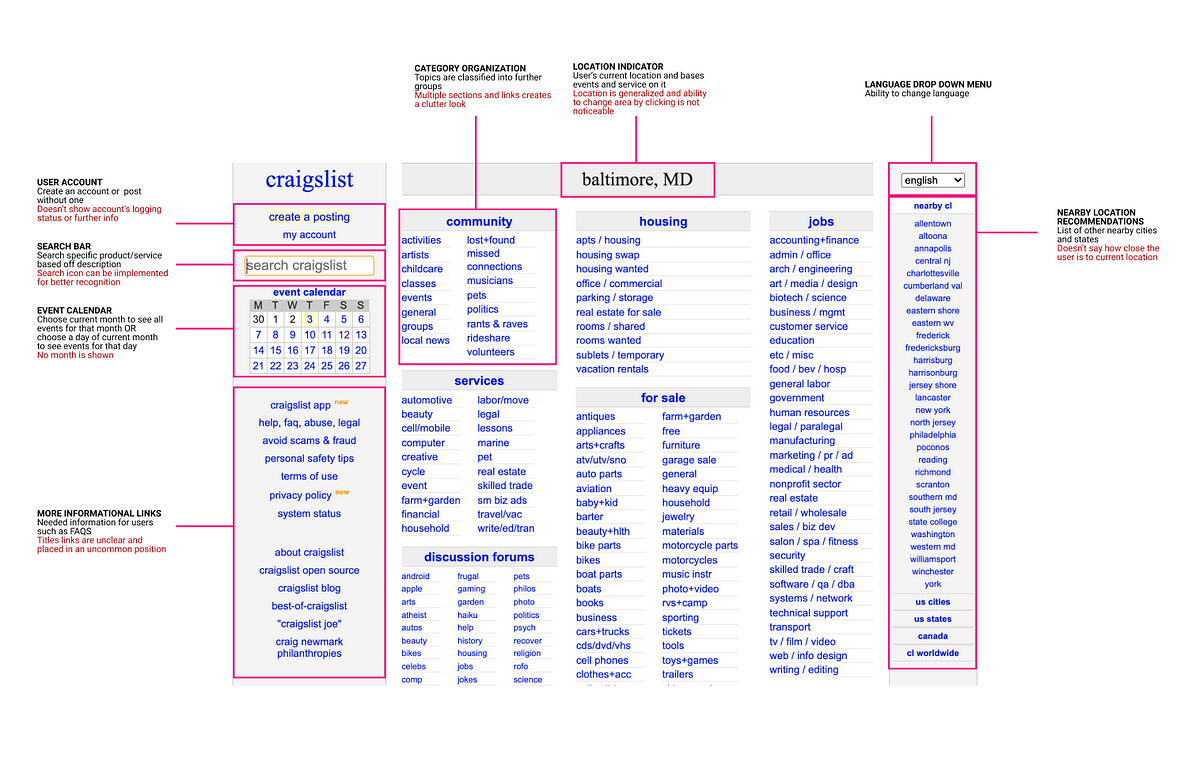The image depicts a complex layout primarily composed of text and boxes, predominantly featuring blue and black text with some elements outlined in red. At the center of the image is a large blue text box with "Craigslist" at the top. The details within this blue box are largely illegible due to the small, blurry font, making the secondary light blue text especially hard to decipher.

Surrounding the central blue text box, there are black and blue text annotations on the left, right, and top of the image. On the left side, black text labels include "user account," "search bar," "event calendar," and "more informational links". Each of these labels is connected to their respective outlined red rectangles by small horizontal lines.

At the very top, black and blue text inputs indicate sections such as "category organization," "location indicator," and "language drop down menu." A small line extends from "category organization" to a red-bordered square labeled "community," though the content within this square is unreadable. Similarly, a line from "location indicator" points down to a highlighted rectangle around "Baltimore MD, Baltimore, Maryland." Below it are sections labeled "housing," "services," "discussion forums," "for sale," and "jobs." The "language drop down menu" has a line leading to a red-bordered rectangle with "English" in a dropdown format. Adjacent to this, another line connects to a segment labeled "nearby location recommendations."

Prominent at the top right of the red-outlined structures are references to categories: "category organization," "location indicator," and "language drop down menu." These help frame the general navigational structure of the diagram. Scattered in this dense layout are references to a "yellow search area," and a possible "calendar" indicated by the days of the week—"M-T-W-T-F-S-S."

While the core structure and some primary labels are readable, much of the finer detail remains indecipherable due to the small, blurry text.